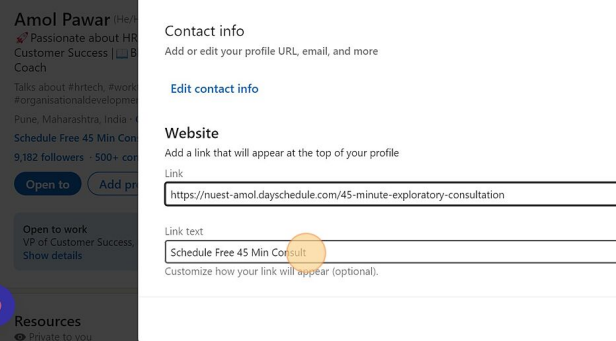This detailed caption describes an image showing a screenshot of a professional's contact information on a website.

---

The image displays a website screenshot featuring the contact information of an individual named Amol Pawar. On the far left side, extending vertically from top to bottom, there is a dark gray sidebar. At the top of this sidebar, the name "Amol Pawar" is prominently displayed. Below the name, a brief description reads, "Passionate about HR, customer success, and [text cut off]." Accompanying this, written in gray letters on the gray background, are hashtags such as "#HRtech," "#work," and "#organizationaldevelopment," indicating the areas of discussion and expertise.

Further down in the sidebar, the location "Pune, Maharashtra, India" is cited, with Maharashtra spelled out as "M-A-H-A-R-A-S-H-T-R-A." Additional information in the sidebar includes: a prompt to "Schedule free 45 minutes" and a note that Amol Pawar has "9,182 followers" and "500+ connections," with the partial text "C-O-R" suggesting "corporations." There is also a blue button labeled "Open to," alongside another label reading "Add PR," hinting at profile addition options. The text "Open to work, VP of customer success, show details" follows, accompanied by a section titled "Resources."

To the right of the dark gray column is a white section of the screen that highlights "Contact Information." This section includes options to "Edit your profile URL," "email," and other contact details. In blue letters, there is a clickable link that reads "Edit contact information." Below this, the page offers an option to add a website link that will appear at the top of the profile. The example link given is "https://nues-t-amol.day-schedule.com/45-minute-exploratory-consultation."

Further customization options are provided, such as including line text like "Schedule free 45-minute consult" and additional options to customize how the link will appear on the profile.